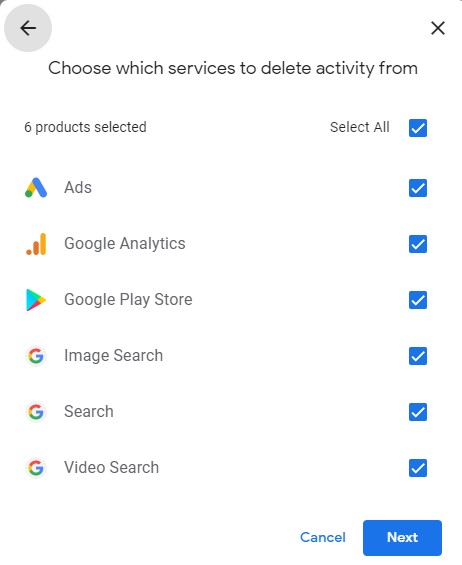The image displays a user interface screen with a white background. In the top left corner, there is a back button represented by a black arrow pointing left, encased in a gray circle. To its right is a small black 'X' icon, serving as an exit button. Centered at the top of the image, the title reads, "Choose Which Services to Delete Activity From."

Below the title is a list of six Android services: Ads, Google Analytics, Google Play Store, Image Search, Search, and Video Search. Each service has a blue checkbox with a white checkmark beside it, indicating selection.

In the bottom right corner of the image are two buttons. The 'Cancel' button is on the left, displayed in blue text without a surrounding color. The 'Next' button is on the right, featuring white text on a blue background. The overall design of the interface is clean and straightforward.